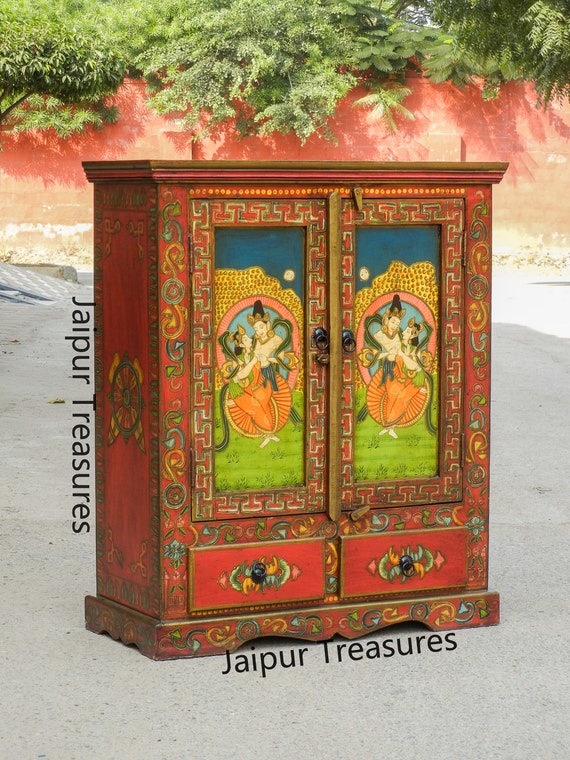This detailed depiction focuses on an ornate, intricately painted item labeled "Jaipur Treasures," possibly a jewelry box, armoire, or cabinet, distinguished by its vibrant Indian-inspired design. The piece, primarily in a darkish red hue with gold trim, boasts rich, detailed artwork on its two tall front doors, which open with knobs and lead to two drawers beneath. The artwork centers around two figures, likely Asian or Indian women, adorned in baggy orange pants, styled with green ponytails, and sitting on grass against a backdrop featuring an orange halo and honeycomb-shaped yellow dots, framed by a blue and pink mosaic-like border. Above this imagery, a moon appears amidst an artificial-looking background of orange walls adorned with green trees. Additionally, a circle sigil in orange and green enhances one side of this captivating piece, adding to the elaborate swirl and square-shaped motifs in an array of vivid colors, underscoring its cultural aesthetic. The surrounding background contrasts with a lilac-gray bottom and peachy top, enhancing the impression that the artwork is possibly a computer-generated drawing rather than a photograph.